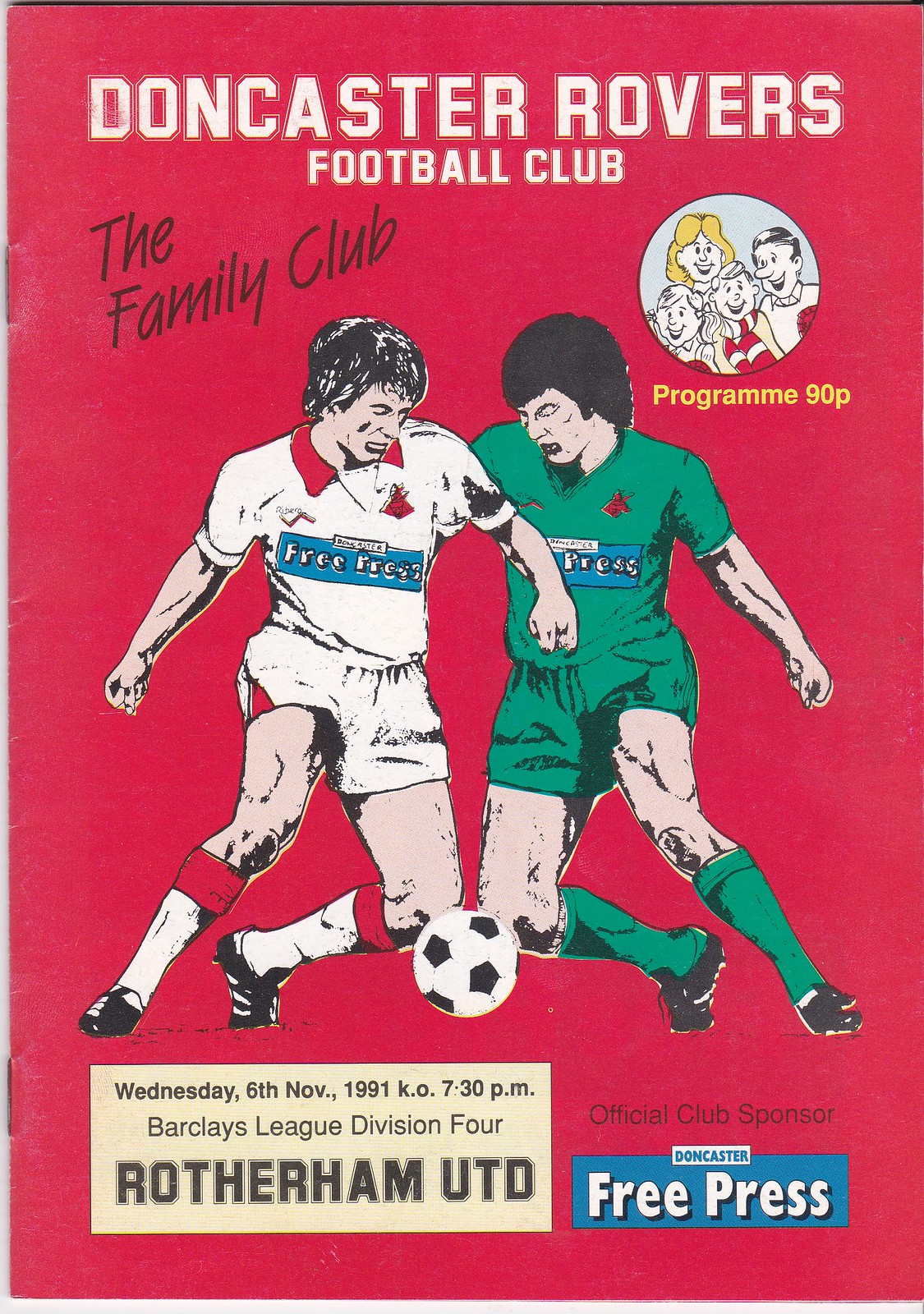This image depicts the front page of a vintage soccer program for Doncaster Rovers Football Club, also referred to as "The Family Club." Dominated by a vibrant red background, the top portion of the cover prominently displays the club's name in large white letters. Just below, in a diagonal, brownish font, it reads "The Family Club." Towards the right side of the cover, there is a circular illustration featuring a cartoon drawing of a family—a man, a woman, and two children—rendered in a light blue font. Below this, in yellow font, it says "Program 90p."

In the center of the page, there are cartoon-style color sketches of two soccer players vying for a ball. The player on the left is depicted in a white jersey with red trim, while the player on the right wears a green jersey with a blue bar across the chest that reads "Free Press," a feature shared by both players' jerseys. 

The bottom section of the cover provides additional details: "Wednesday, 6th November, 1991, KO 7.30 p.m. Barclays League Division IV, Rotherham UTD." To the right, it notes that the "Official Club Sponsor" is "Doncaster Free Press." The image also shows staples on the left-hand side, suggesting a magazine-like binding. The overall aesthetic is vividly colored yet maintains a vintage feel, typical of soccer programs from that era.